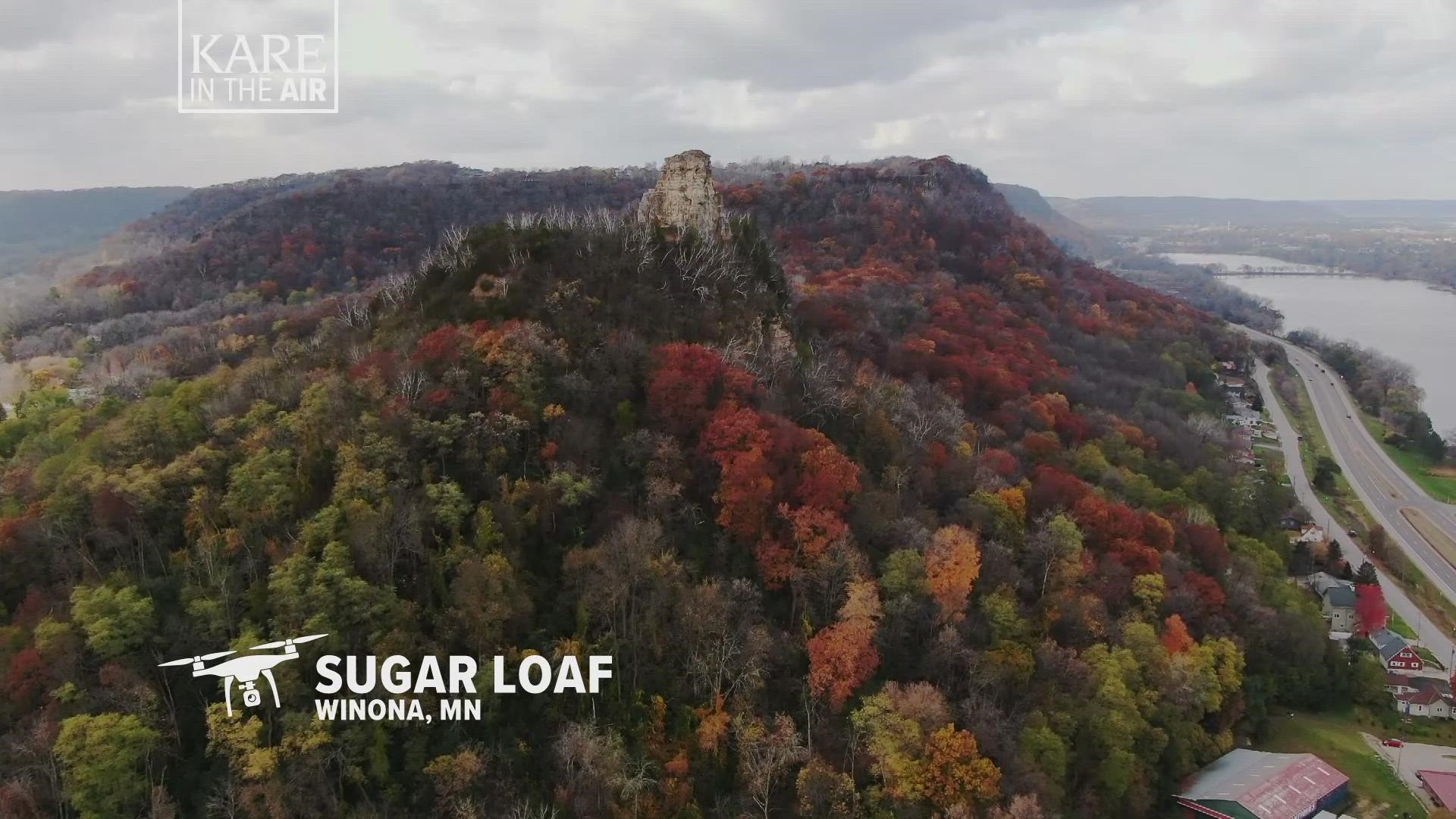This aerial photograph, presumably an advertisement in landscape mode, beautifully captures the vibrant fall foliage surrounding Sugarloaf in Winona, Minnesota. Dominated by a dramatic dark gray sky filled with stormy clouds, the image's top left corner features a white logo that reads "KARE in the air," stylized with a capital K-A-R-E and bordered by a mostly white square. The scene below is a canvas of autumnal splendor, showcasing a forest with fluffy trees in vivid hues of green, red, and pink. In the bottom left corner, a white drone icon alongside the text "Sugarloaf" clearly identifies the location as Winona, MN. The right-hand side of the image reveals a serene neighborhood complete with green grasslands, a parking lot, and distinctive red roofs. A road winds from the right edge towards the center, leading to a broad, grayish river and additional trees beyond. The landscape is punctuated by a central tan structure resembling a castle that stands out against the colorful foliage, further enhancing the picturesque quality of the fall scene.